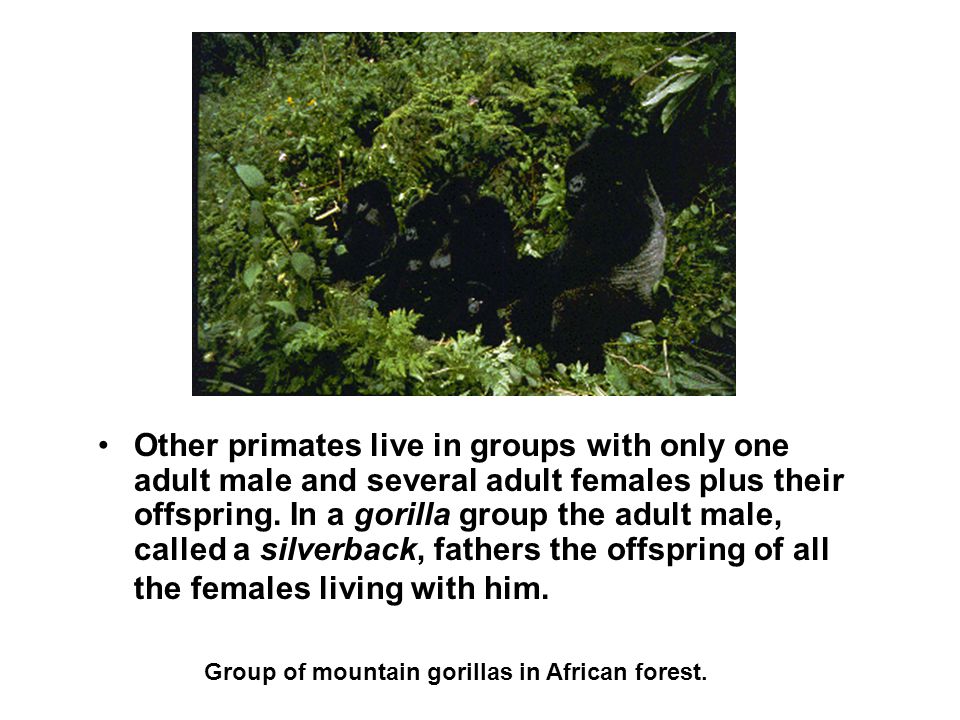This color photograph captures a serene moment in an African forest with a group of mountain gorillas. In the lush green environment filled with ferns and wide-leaf plants, four gorillas are seen sitting amidst the dense foliage. On the left, three smaller gorillas, possibly youngsters, sit in a row looking towards the left. To their right, a larger adult male gorilla, with distinctive gray hair on his back, also gazes leftward. This adult male is a silverback, identifiable by the gray coloring on his back, and he fathers the offspring of all the females within his group. The dense jungle setting blends the gorillas into their surroundings, making them a little hard to distinguish at first. The text below the image provides further insight: "Other primates live in groups with only one adult male and several adult females, plus their offspring. In a gorilla group, the adult male, called a silverback, fathers the offspring of all the females living with him." Also included is the caption: "A group of mountain gorillas in African forest."